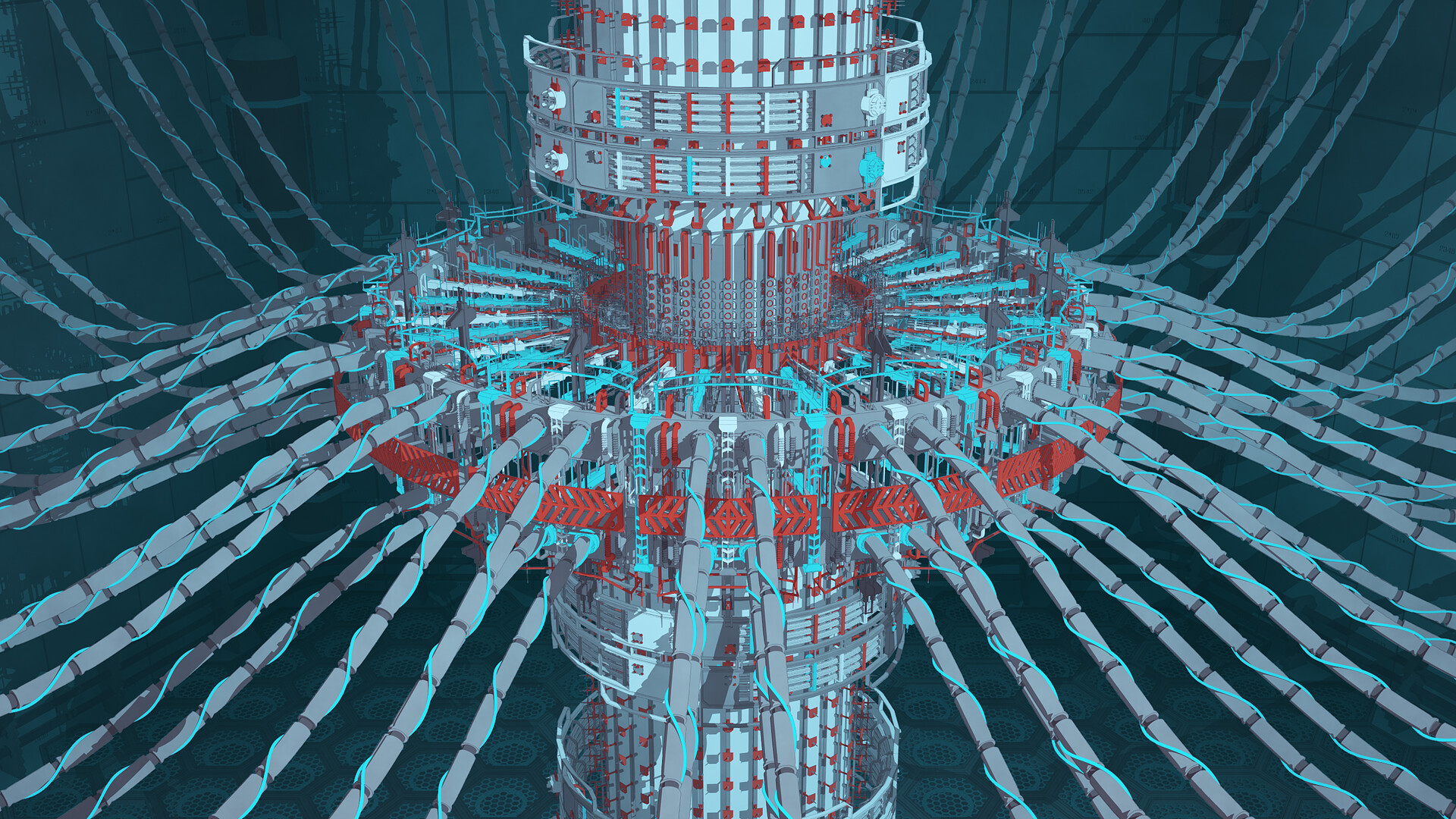The image depicts a highly detailed, computer-generated model of an immense and intricate piece of machinery. At the center of this machinery is a colossal cylinder, primarily colored in shades of gray with accents of white, red, and blue. Several circular metal rings, resembling platforms or balconies, encircle the cylinder at multiple levels, suggesting areas for maintenance or observation. Extending from these metal rings, a complex network of cables and pipes in gray and light blue fan outwards, intertwining and stretching horizontally across the image, creating a sense of connectivity and industrial complexity.

The middle section of the cylinder features a notable metal circle that extends outward, giving the appearance of a large gear or crank, implying that this section might rotate or have a specific mechanical function. The overall scene is set against a muted blue background with a contrasting dark green wall that appears to frame the machinery, enhancing the sense of depth and dimensionality. Red accents are sporadically placed throughout the device, adding a striking visual contrast to the predominantly cool color palette. The environment evokes an industrial or scientific setting, emphasizing the sophistication and complexity of the apparatus depicted.